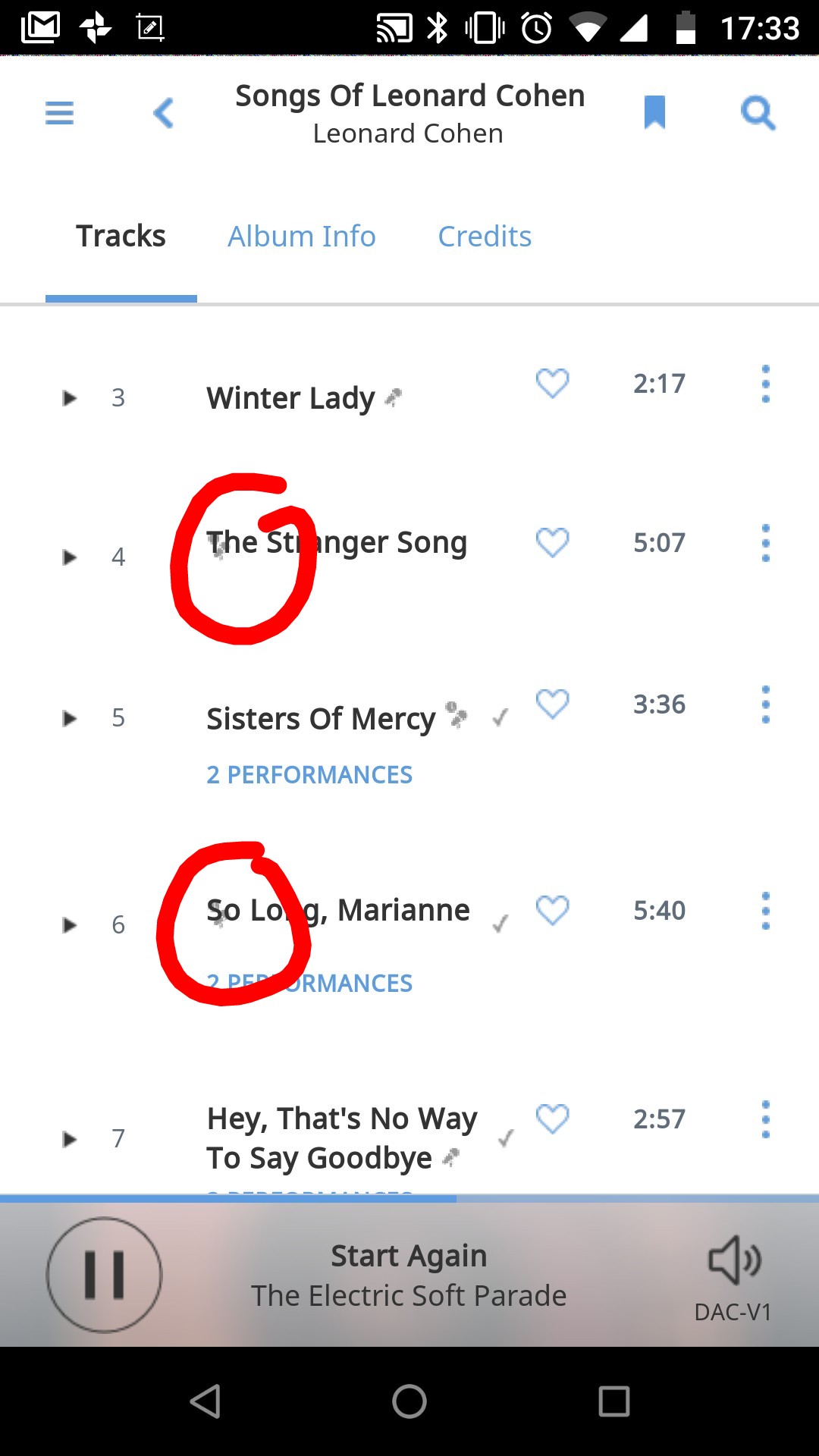This description provides a comprehensive view of an Android smartphone screenshot featuring a music app. Here’s the cleaned-up and detailed caption: 

---

This screenshot, taken from an Android smartphone, showcases a music app currently displaying Leonard Cohen's album "Songs of Leonard Cohen." At the very top, a black status bar indicates the time as 17:33 (5:33 PM). The battery icon shows approximately 50% charge, with both strong Wi-Fi and cellular network signals. Additional icons indicate an active alarm, Bluetooth connection, and Gmail notifications, though some icons are unclear.

The app interface is segmented into three tabs at the top: "Tracks," "Album Info," and "Credits." The "Tracks" tab is currently selected, displaying a list of songs from the album. Visible tracks include: 
1. Winter Lady
2. The Stranger's Song
3. Sisters of Mercy
4. So Long, Marianne
5. Hey, That's No Way to Say Goodbye

Significantly, parts of "The Stranger's Song" and "So Long, Marianne" are marked with red circles around the initial letters ("T-H-E-S-T" and "S-O-L-O"), likely highlighting them for emphasis.

At the bottom of the screen, another section reveals that the song "Start Again" by The Electric Soft Parade is currently playing. There are options to pause the song or adjust the sound via the "DAC-V1" icon featuring a speaker with sound waves.

The very bottom black bar contains the navigational buttons typical of an Android device: the menu button, the home button, and others, ensuring easy navigation.

This detailed screenshot provides an intricate look at both the music app interface and the Android device functionality.